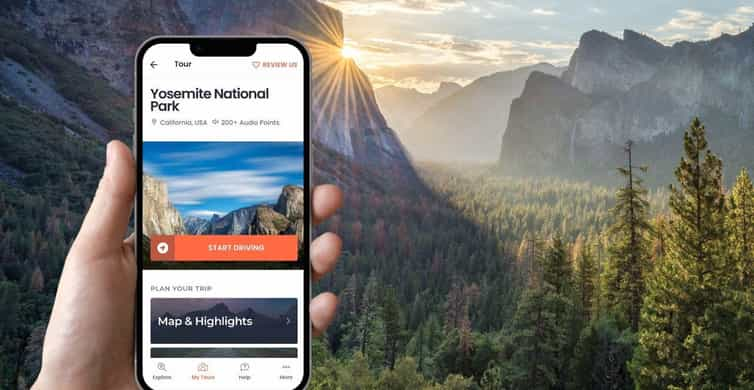The digitally created image appears to be an advertisement for Yosemite National Park, but it has an oddly manipulated look that detracts from its authenticity. The background ostensibly depicts a breathtaking park vista, yet it seems artificial, which is ironic given Yosemite's natural beauty. The scene showcases a majestic valley blanketed with towering pine trees, flanked on both sides by colossal gray stone mountain ranges. The sun is partially obscured by the mountain on the left, casting dramatic light rays that scatter as if viewed through a glass lens.

Dominating the foreground is a conspicuously photoshopped image of a man's hand holding a cell phone, which occupies a significant portion of the picture. The phone's screen displays the Yosemite National Park website, prominently featuring information like "California, USA" along with various navigational options, such as directions to the park. The overall effect, while aimed at promoting Yosemite, suffers from an unnatural composition that diminishes the genuine allure of the iconic landscape.